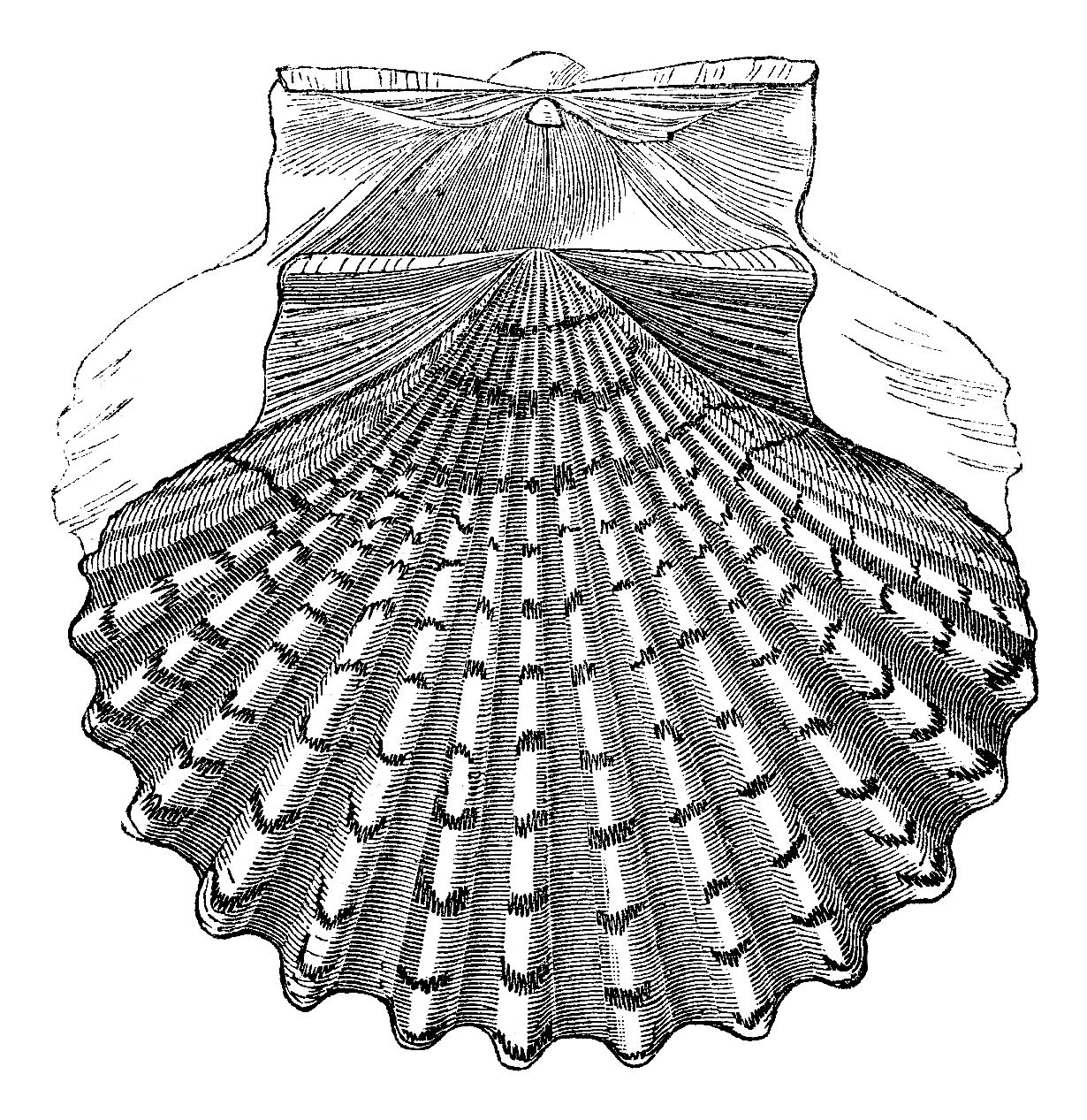The image is a detailed sketch featuring an abstract design predominantly rendered in black, white, and shades of gray. At the center of the composition, which serves as the focal point, the design resembles an upside-down seashell or a folded hand fan with a series of radiating, ripple-like ridges. These ridges are accentuated by vertical white stripes separating each black line, creating a sense of depth and texture. The sketch is free of any text and is characterized by several spokes or ridge lines emanating from the central apex, spreading downward. Toward the top of the image, there appears to be an ambiguous structure resembling a bow or perhaps the upper part of a dress, adding an element of intrigue and complexity. The entire scene gives the impression of an intricate, hand-drawn design, possibly created with pencil or pen, showcasing a harmonious blend of abstract elements and suggestive shapes.